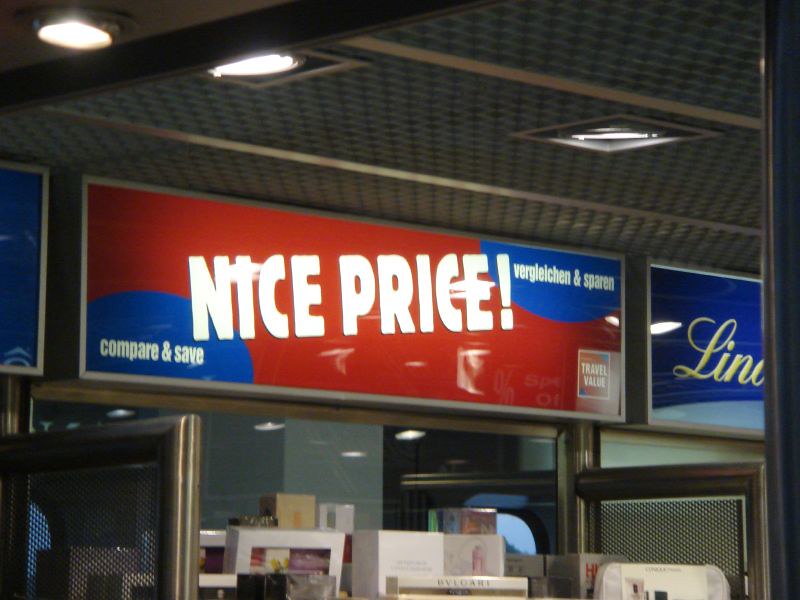This photograph captures a storefront display viewed from the outside. The centerpiece consists of various boxes arranged neatly, including a mix of white boxes, white and gold-colored boxes, and a conspicuous gold-colored box. The contents of these boxes are indistinguishable due to the distance from the camera. Framing the display are black metal frames with a black mesh insert on either side, giving the scene a structured and industrial aesthetic.

Above the display boxes hangs a horizontal rectangular sign, predominantly red with blue corners. The middle section of the sign contains the phrase "NICE PRICE!" in bold white letters, suggesting a promotional offer. The bottom right of the sign features the term "Travel Value," while the bottom left corner showcases a blue circle with the text "Compare and Save," emphasizing the store's competitive pricing.